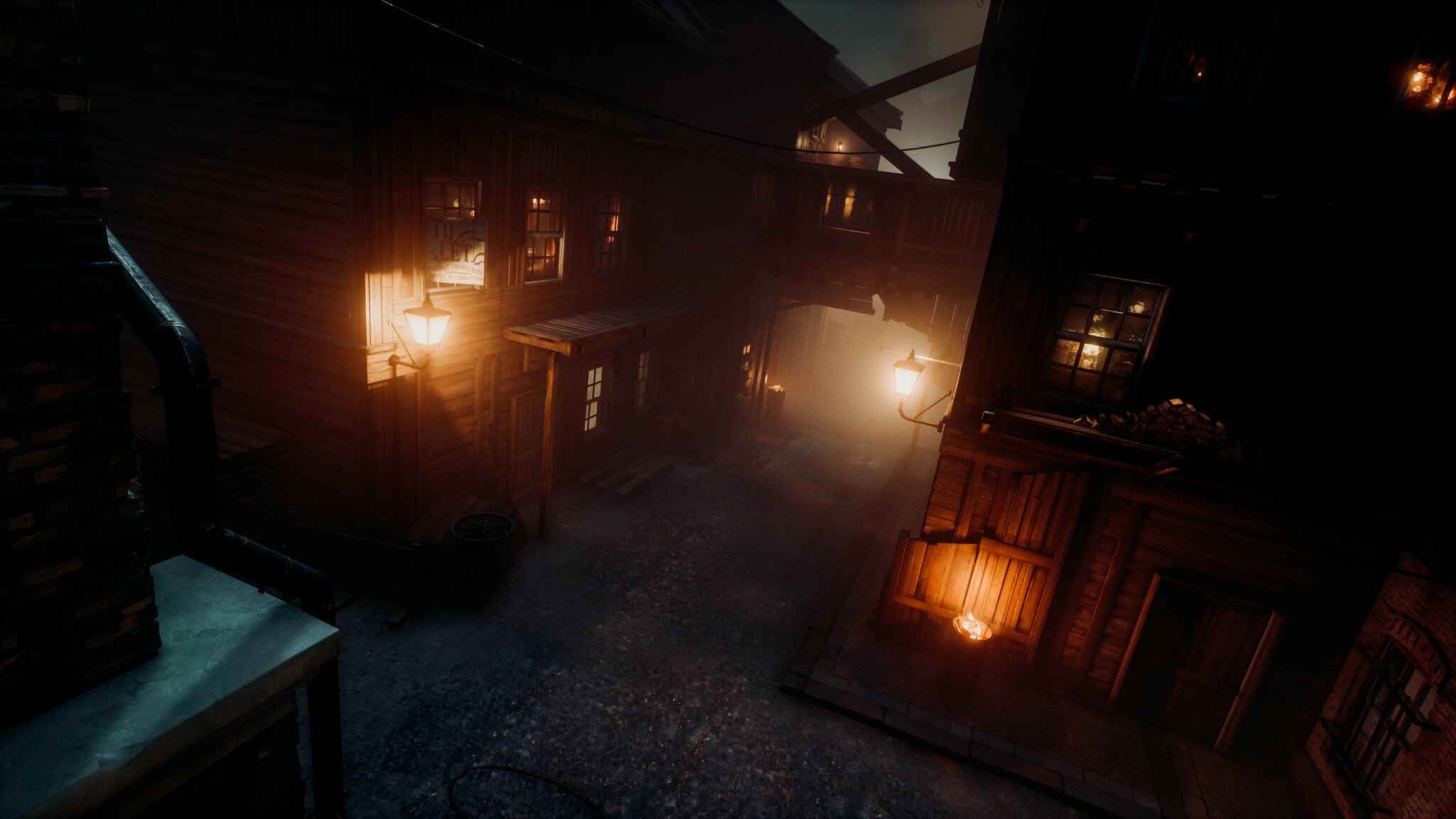The image depicts a dark and atmospheric scene, seemingly from a video game or a film, set in an old, narrow alleyway at nighttime. The alley is flanked by two shabby, two-story wooden buildings with elements of stone construction here and there. The cobblestone street running through the alley glistens, suggesting a damp, rainy environment, which adds to the overall haziness.

Both buildings exhibit multiple illuminated windows, casting a warm glow in the otherwise misty and shadowy setting. The building on the left features a prominent white sign on the second floor that reads "Tillette." This building has a roof over the door on the ground floor, with three windows on the upper level and two windows below. An exterior lantern adds to the sparse lighting providing visibility in the dimly lit alley.

Connecting the upper floors of the buildings is a wooden bridge or walkway, suspended above the cobblestone path. The building on the right showcases a second-story window with a stack of firewood nearby, while the ground floor sports double doors and a window protected by metal bars.

In the left corner of the image, partly obscured by the darkness, stands a statue that is difficult to discern, adding a mysterious element to the scene. Overall, this image captures the essence of an eerie, rain-soaked night in a vintage, possibly Western-style town.